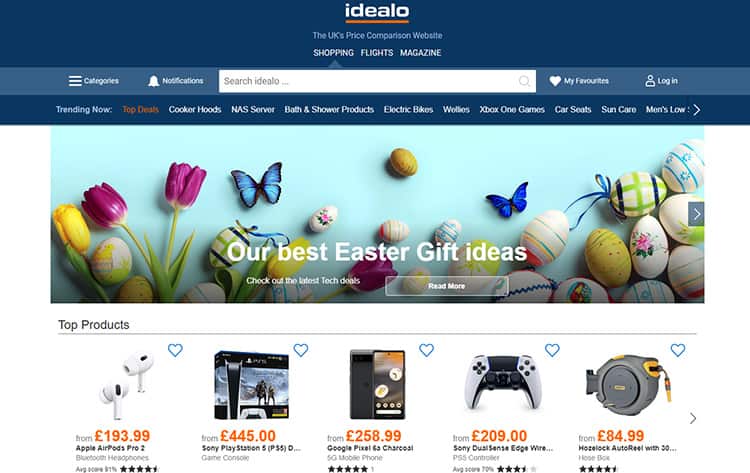The webpage appears to be a product-oriented website with a focus on price comparisons, likely named IDEALO based on the logo. Here is a detailed description of its layout and features:

---

The header of the website prominently displays the logo "IDEALO" in bold white letters, accompanied by an orange horizontal line beneath it. Below the logo, the text "the UK's price comparison website" is displayed in a light blue font against a darker blue background.

Immediately below the header, there is a blue-gray navigation bar with various menu options. On the left side, three horizontal lines indicate a menu for categories, followed by a bell icon for notifications. In the center, there is a white search box with placeholder text "Search IDEALO..." and a magnifying glass icon indicating the search functionality. To the right of the search bar, there is a heart icon labeled "My favorites" and a login option represented by a person icon.

Directly below this navigation segment, the site features a "Trend Now" section with the title "Top Deals" in orange text. The section includes a carousel of trending categories such as Cooker Hoods, NAS servers, Bath and Shower products, something from But Tronic (text is hard to read), X1 games, Car Seats, Sun Care, and Men's products. Some text may be truncated due to resolution issues, followed by a right-direction arrow indicating additional options.

A hero image is located below the "Trends" section, highlighting "Our Best Easter Gift Ideas" with a prompt that says, "Check out." The accompanying button is transparent with a white border and white text that says "Read More."

Continuing down the page, there is a "Top Products" section showcasing five different items. Each product is displayed with its image, name, star rating, and price listed in pounds (£).

---

In summary, the website layout and elements suggest a structured and user-friendly interface designed to help users find the best deals and compare prices across various product categories.